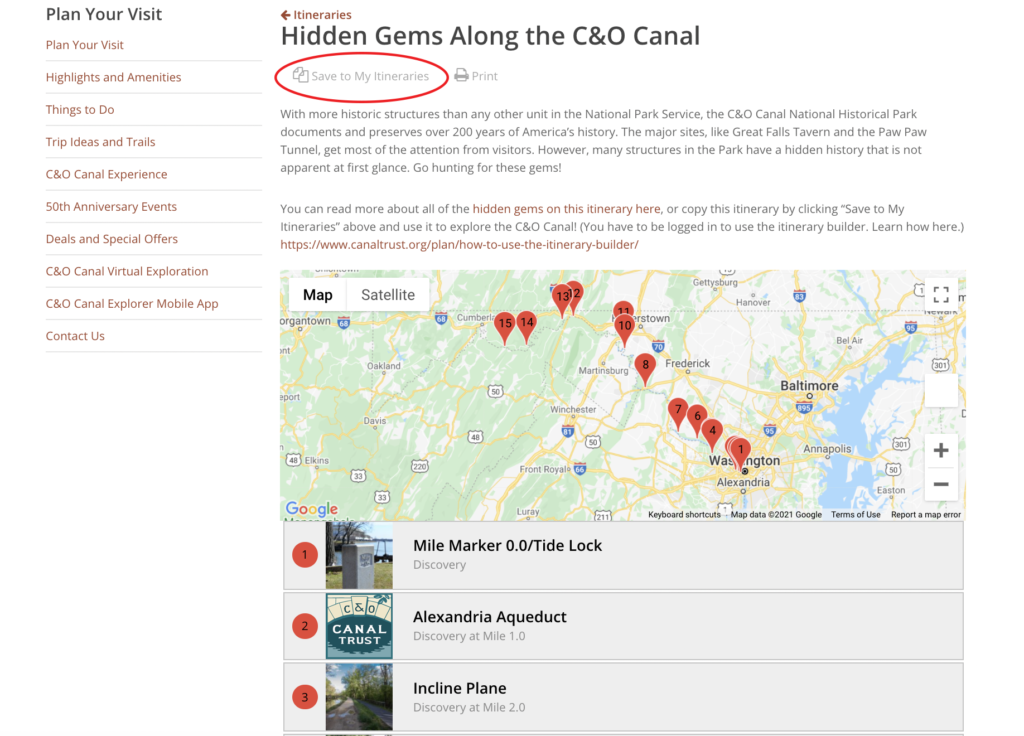**Explore the C&O Canal National Historic Park - Plan Your Visit**

The image features a detailed guide for planning your visit to the C&O Canal National Historic Park. The guide is presented in a sleek design with black lettering and sections of the menu highlighted in orange hyperlinks. Key sections include "Plan Your Visit," "Highlights and Amenities," "Things to Do," "Trip Ideas," "Trails," "C&O Canal Experience," "50th Anniversary," "Special Offers," "C&O Canal Virtual Exploration," "C&O Canal Explore Mobile App," and "Contact Us." 

At the top, there's a section for "Itineraries" with an option to "Save to My Itineraries" that is circled for emphasis. This tool helps users to meticulously plan their visit, focusing on the C&O Canal's rich history and attractions. Alongside key destinations like Great Falls Tavern and the Paw Paw Tunnel, visitors are encouraged to uncover the park's numerous hidden historical gems. 

By saving itineraries, visitors can create personalized tours of the C&O Canal, provided they are logged into the website. There's a convenient link to learn how to use the itinerary builder: [How to Use Itinerary Builder](https://www.canaltrust.org/plan/how-to-use-itinerary-builder).

Displayed on the page is a map highlighting key areas around Washington, D.C., near Alexandria, and Baltimore - landmarks close to the canal trailheads such as Mile Marker 00 at Tidal Lock, Alexandria Aqueduct, and Incline Plane.

Experience the park's blend of natural beauty and historical significance by accessing the comprehensive visitor guide to optimize your exploration of the C&O Canal National Historic Park.